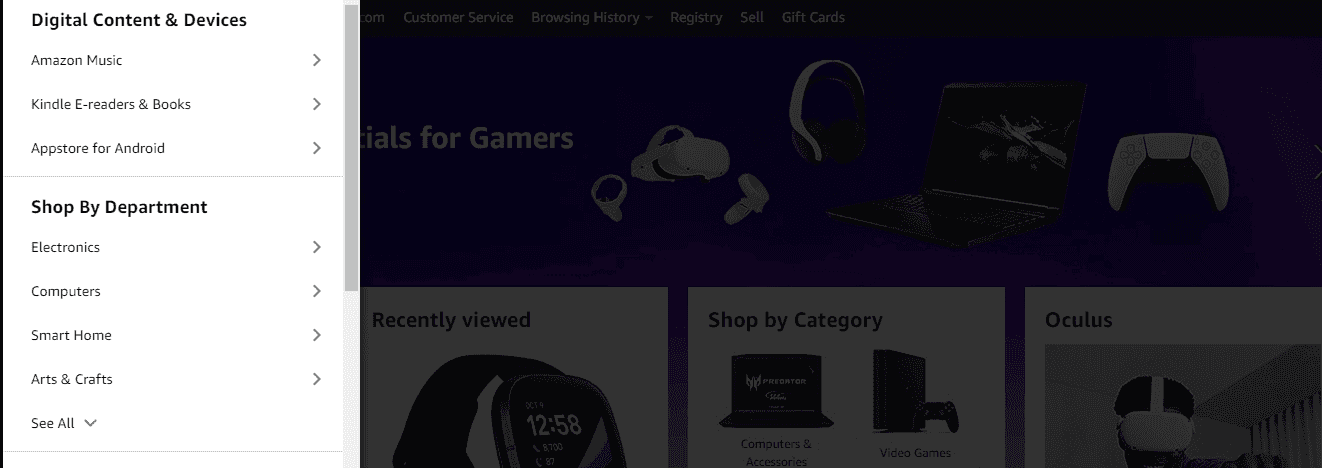The image displays a snapshot of the Amazon shopping website, specifically showcasing a section dedicated to gaming and gaming-related products. On the left-hand side of the page, a menu tab is open against a white background, presenting two main categories with multiple menu items.

The first category, "Digital Content and Devices," includes three menu items:
1. Amazon Music
2. Kindle E-Readers and Books
3. Amazon Appstore for Android

The second category, "Shop by Department," features several options:
1. Electronics
2. Computers
3. Smart Home
4. Arts and Crafts
5. See All

To the right of this menu, there is a large, dark box, almost black, containing a prominently featured banner. The banner is designed with a darker hue and showcases various gaming products aimed at gamers, including a virtual reality headset, headphones, a gaming laptop, and a gaming controller.

Beneath this banner, there are three additional sections with the following headings:
1. "Recently Viewed" – displaying an image of a partially cropped smartwatch, resembling an iWatch.
2. "Shop by Category" – offering two options: Computers and Accessories, and Video Games.
3. "Oculus" – depicting an individual wearing a virtual reality headset.

Overall, the webpage is visually organized to guide users through different gaming products, recent views, and categorized shopping options.